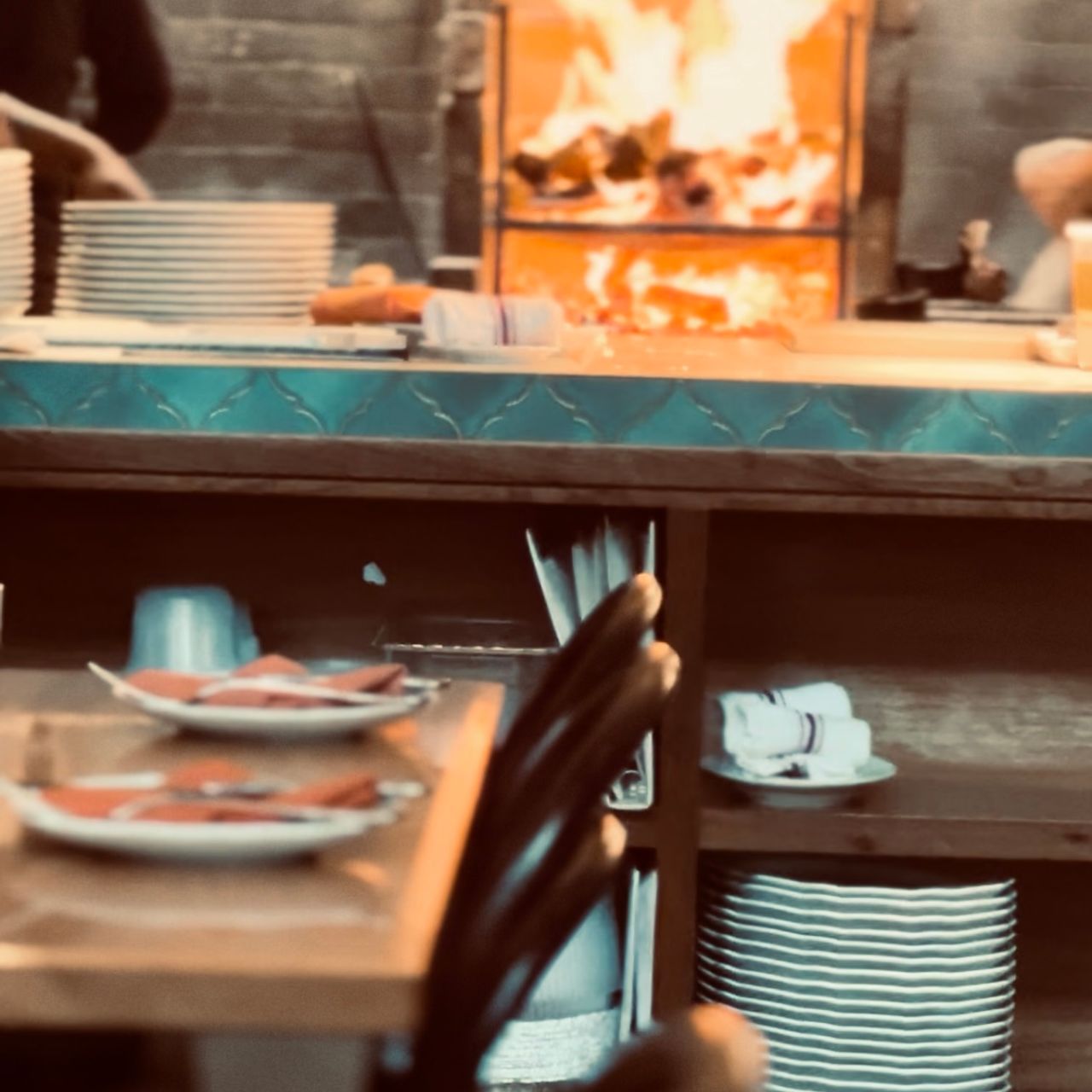The image captures a cozy restaurant dining area with a strong emphasis on its rustic, inviting ambiance. In the central background, a large, roaring fireplace set into a gray stone wall provides a warm and comforting glow. A countertop separates the dining area from the kitchen, with a stack of white dishes resting neatly atop it. The area beneath the countertop features dark wooden shelves, holding various dishes. A table in the bottom left corner is decked with unused place settings, suggesting readiness for incoming guests. Additional details include visible arms clothed in black, belonging to a person partially in frame in the upper left corner, adding a subtle human presence. The overall scene showcases an organized and welcoming environment, reminiscent of a classic diner, where the carefully arranged plates and utensils highlight the restaurant's preparedness and attention to detail.